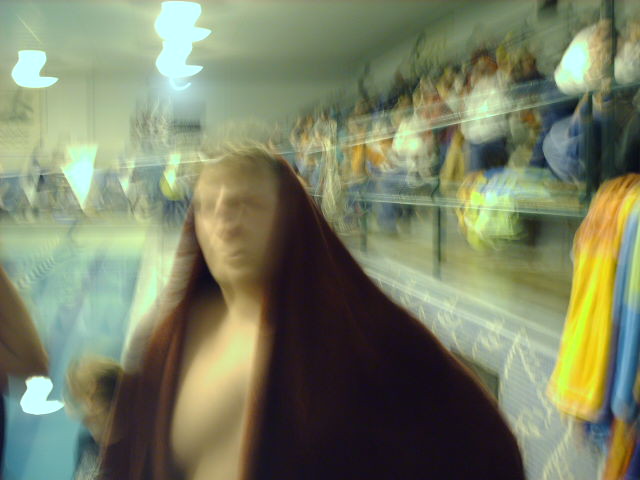The photograph appears to have been taken with significant camera shake, resulting in a highly blurred image that is difficult to decipher. At the bottom of the picture, there are indistinct blue and brown shapes. The lighting in the image consists of streaked, blurred patterns that resemble faded brushstrokes across the frame. In the center of the image stands a bald man, looking directly at the camera. He is partially draped in what seems to be a brown cloak or robe, covering half of his head and body. The background features blurred objects and streaked lights, including green, blue, and white hues, as well as what appears to be blurred rails. The overall effect is a chaotic mix of colors and shapes surrounding the central figure.